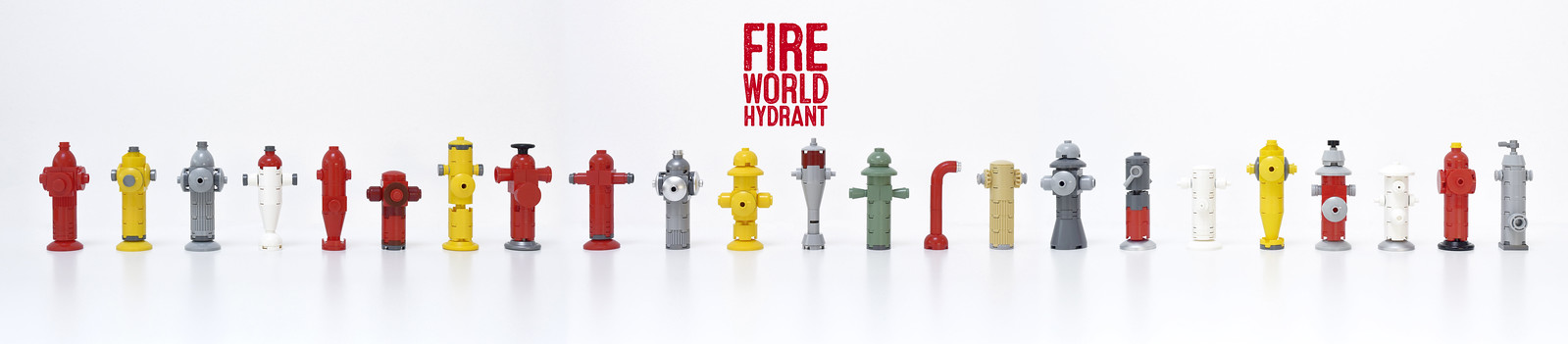The image is a horizontally rectangular frame with a white background, featuring an array of miniature fire hydrants from around the world. At the center, in bold capital letters in three lines, it says "FIRE WORLD HYDRANT" with the word "FIRE" being the largest, followed by "WORLD" in a slightly smaller font, and "HYDRANT" in the smallest. The hydrants are meticulously lined up from left to right, showcasing a variety of styles, shapes, and colors. The lineup includes red, yellow, gray, green, white, brown, blue, and silver hydrants, with some having multicolored designs such as white with red tops or red with silver bottoms. Subtle shadows indicate that the image is lit from behind, adding depth to the scene. The detailed arrangement highlights the diversity of fire hydrants globally, with each uniquely colored and styled hydrant standing out against the stark white background.